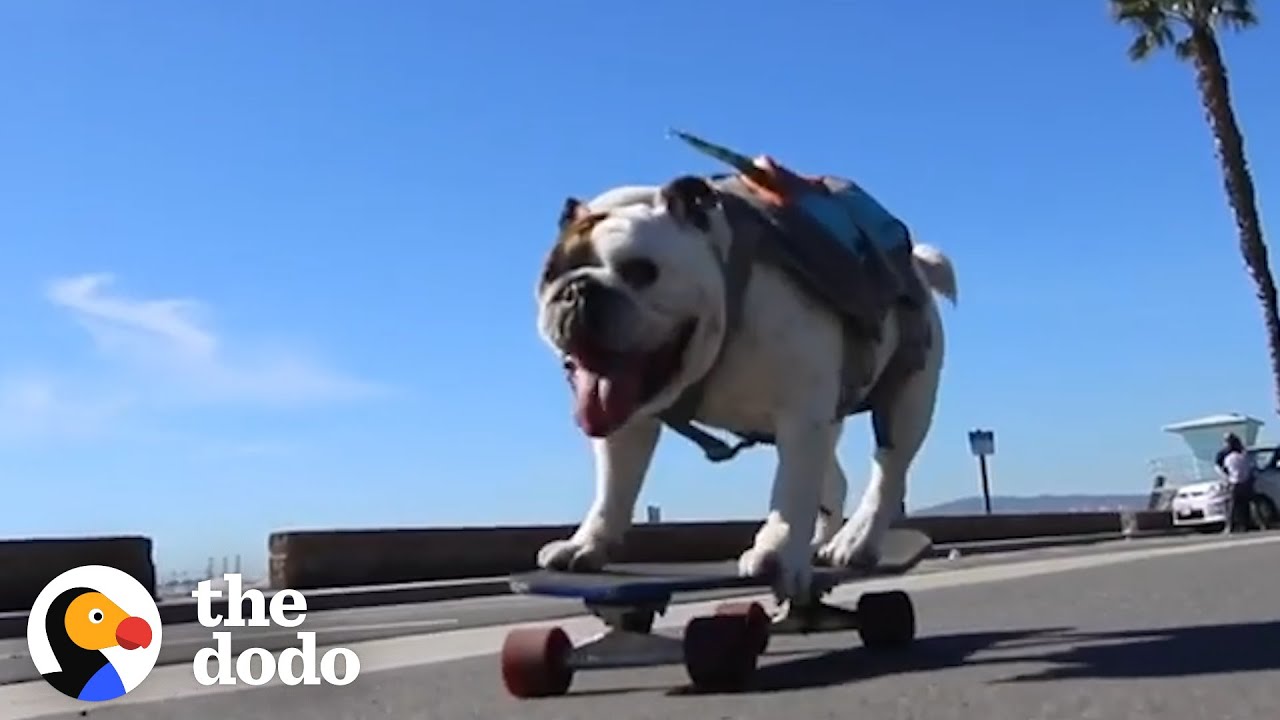This captivating photograph captures a memorable outdoor scene on a sunny day under a bright blue sky with a small, puffy white cloud. The main focus is a joyful bulldog, predominantly white with a distinctive brown patch over one eye, riding a blue skateboard with red wheels. The bulldog is energetically smiling at the camera with its tongue playfully hanging out and appears to be carrying a backpack or a harness strapped around its back. Situated on a paved road, the image also features a parked car with its hood up and a couple of people standing beside it in the distance. Enhancing the tropical vibe, a tall palm tree rises near the car with its fronds extending upward. In the bottom left corner of the image, the logo for The Dodo is visible, depicting a colorful bird with a black head, orange face, and red beak, marking the photograph's connection to the popular media brand. The distant mountains suggest a picturesque location, possibly Southern California, adding to the overall cheerful and adventurous ambiance of the photo.